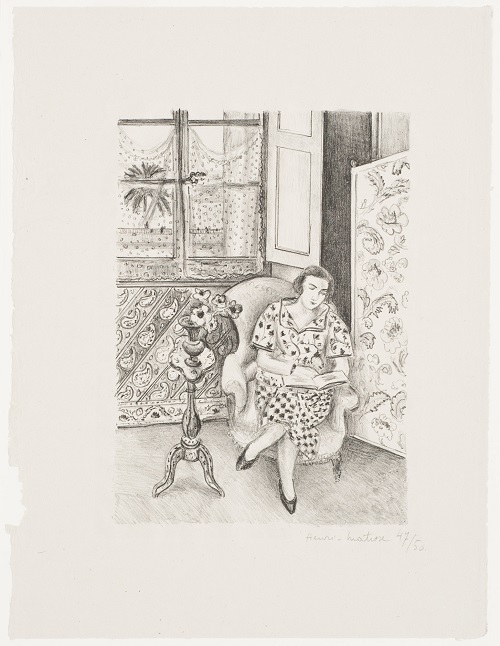This detailed drawing captures a serene, black-and-white scene of a woman sitting elegantly in an armchair, engrossed in a book. The antiquated-quality paper, cream-colored and weathered with ripped edges, adds a vintage touch. Surrounding the central artwork is a one to one and a half inch beige matting, complemented by a white frame. The woman, dressed in an old-fashioned, flowery dress and black shoes, sits gracefully with her legs crossed. Behind her, an open window with polka-dotted curtains and white shutters lets in light. To her left, an ornate dressing screen acts as a room divider, while to her right, a small antique table holds a flower. The wallpaper adorned with flower motifs further enhances the room’s charm. The scene exudes tranquility and elegance, reminiscent of a bygone era. Below the drawing lies an artist's signature and potentially a print number, though it remains indecipherable.